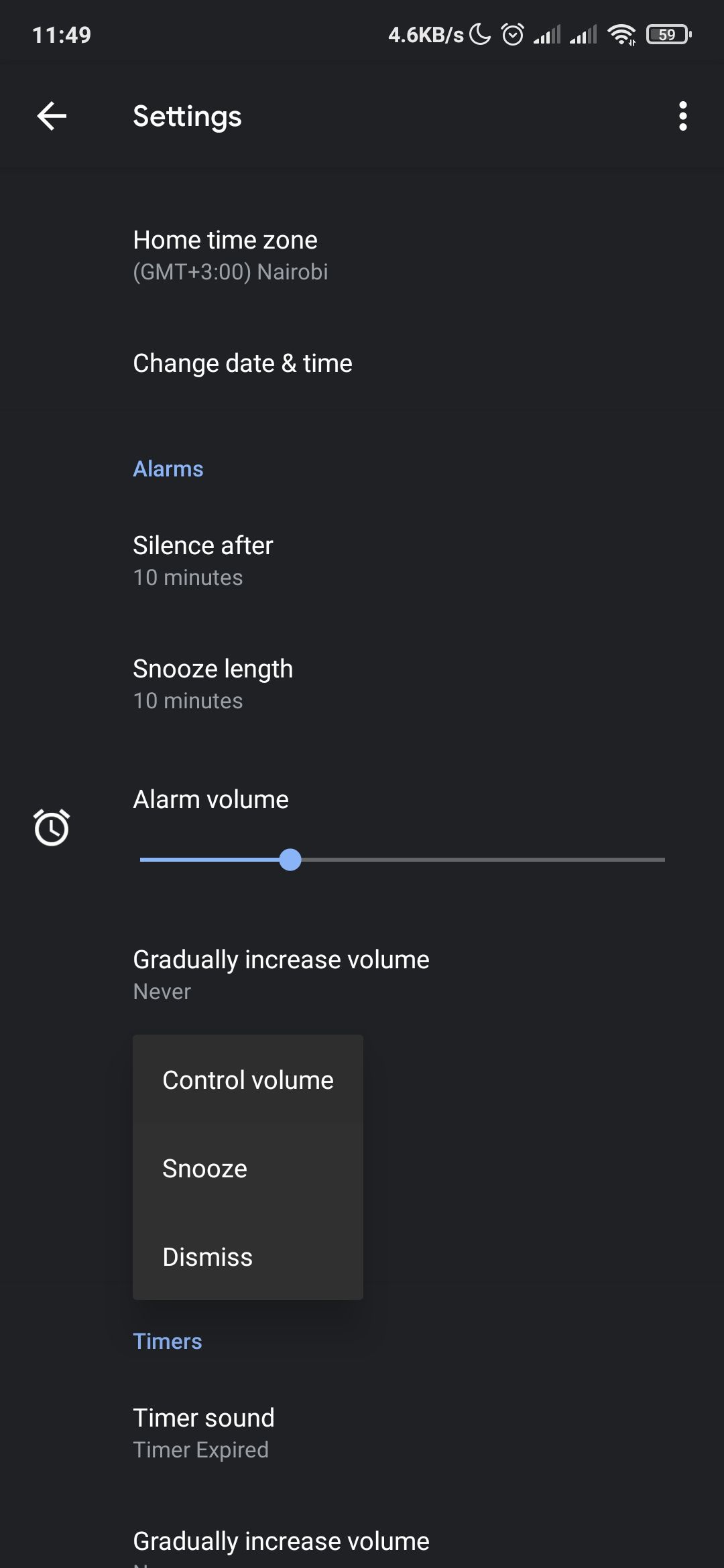The image displays a detailed view of a smartphone interface within the alarm settings menu. The top status bar indicates various system details: 

- Signal strength showing 3 out of 5 bars
- Full Wi-Fi connectivity
- A battery level at 59%
- Time is set to the GSM+3 timezone, specifically Nairobi.

Below this status bar are several sections including options to change the date and time, set alarms, and manage alarm settings. Various user controls are visible including:

- An option to silence the alarm after 10 minutes
- An adjustable alarm volume setting that can gradually increase the volume
- Controls for snooze and dismiss functions

The interface features a predominantly gray background with contrasting blue and white texts. "Timers" is highlighted in blue text, while "Timer Sound" and "Timer expired" are in white and gray texts, respectively. 

Overall, the layout conveys a functional design focused on user customization and control over alarm settings.